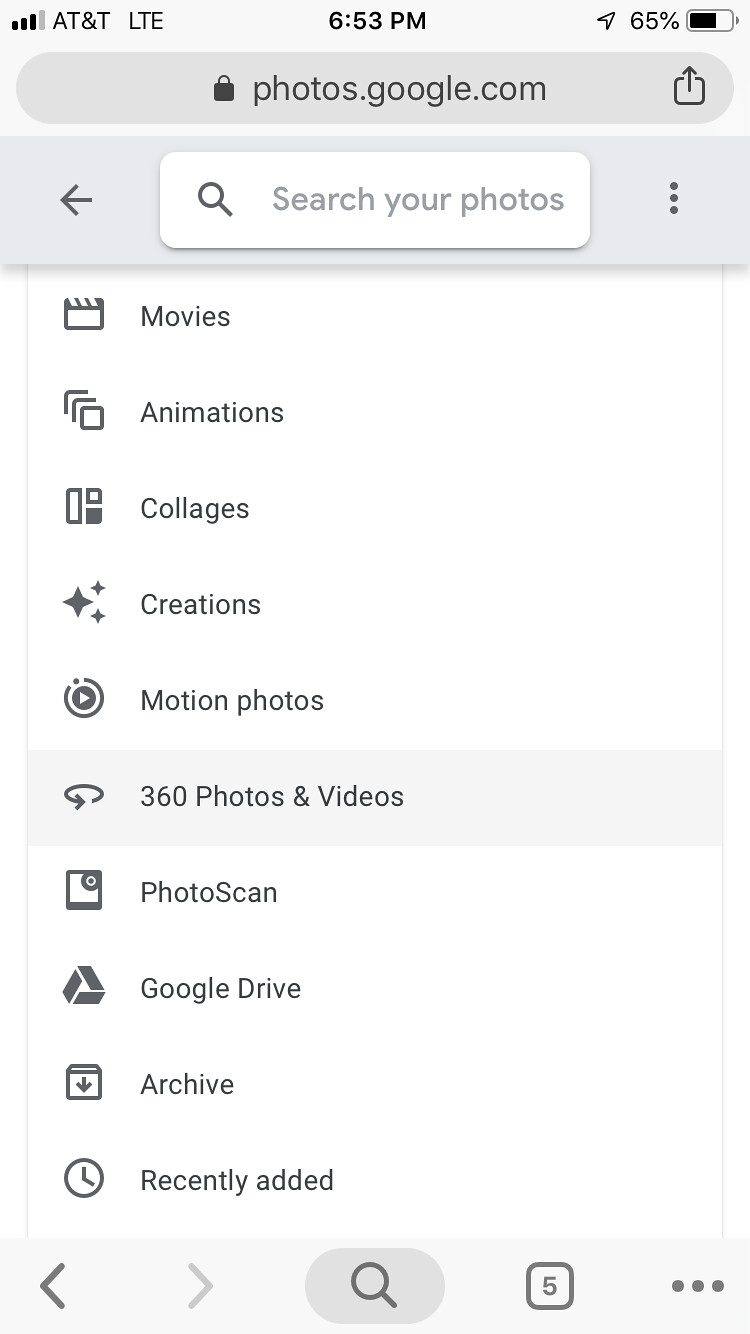The image displays a screenshot of the Google Photos app interface on an iPhone. 

At the very top, the status bar indicates the following details:
- Website: photos.google.com
- Lock symbol
- Mobile carrier: AT&T
- Connection type: LTE
- Time: 6:53 PM
- Battery: 65% with charging symbol
- Three-bar signal strength icon

Below the status bar, the app interface is organized with various multimedia categories. From top left to bottom left, the icons and text visible include:
- Movies
- Animations
- Collages
- Creations
- Motion Photos
- 360 Photos and Videos
- Photo Scan
- Google Drive
- Archive
- Recently Added

At the bottom of the screen, there is the navigation bar with several icons:
- Bottom left: Left arrow (to go back) and right arrow (to go forward)
- Magnifying glass (search function)
- Bottom right: Number five representing the tabs open and the three-dot settings icon

Additionally, at the top of the app interface:
- Arrow pointing to the left (likely to go back)
- Search bar labeled "Search your photos"
- Three dots (more options)
- Share button icon

Overall, the screenshot provides a comprehensive view of the Google Photos app's interface on an iPhone, detailing the status bar, multimedia categories, and navigation options.